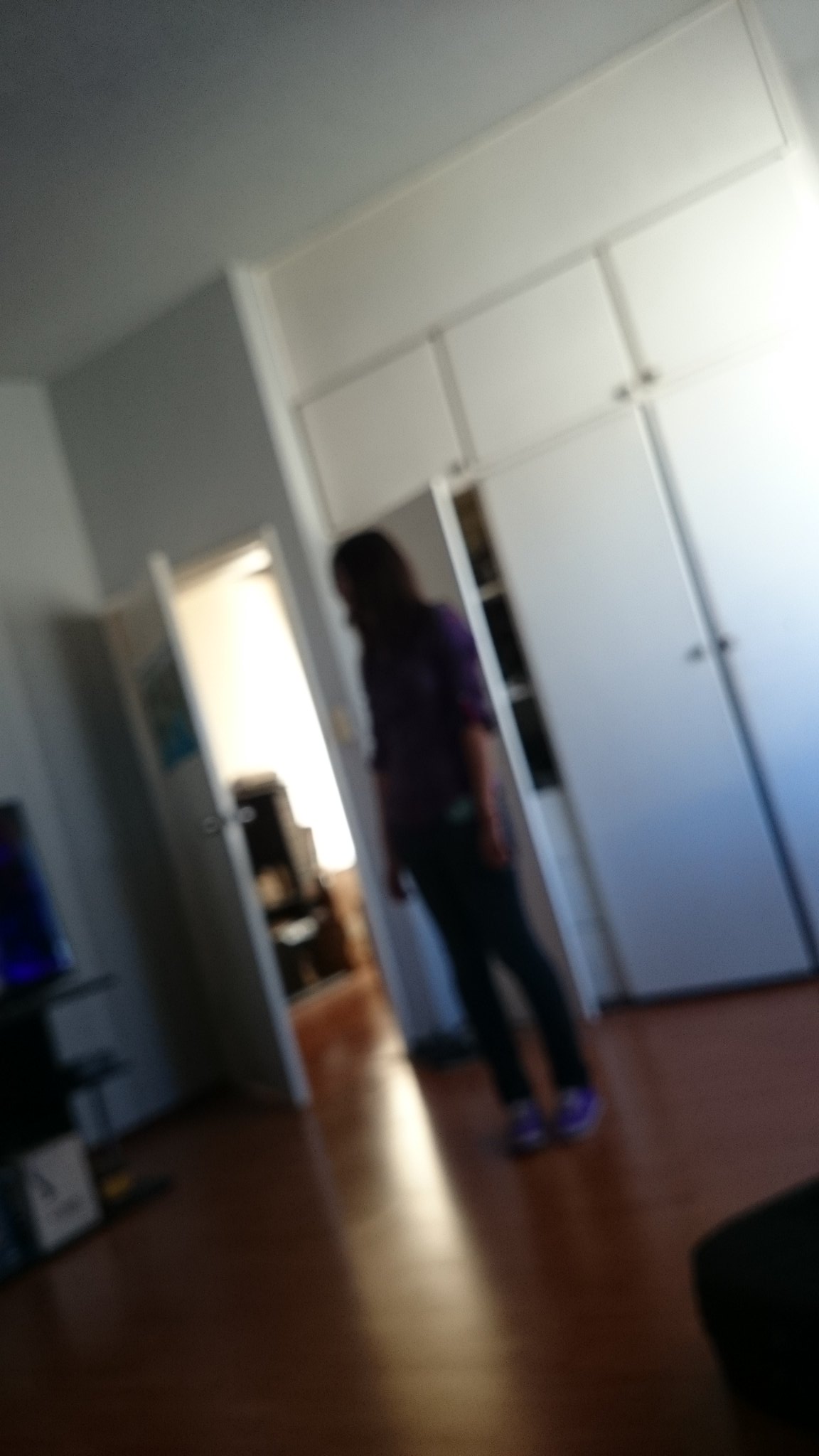This out-of-focus image depicts a person standing in what seems to be a large kitchen with prominent white cabinets and a shiny medium to dark brown hardwood floor. The person appears to be a girl or woman with long brown hair, dressed in blue jeans, purple sneakers or shoes, and a button-up shirt that might be flannel, with the sleeves rolled up. The backdrop includes white walls and a significant number of white cabinets, lined up in three large sections with smaller cabinets above them. On the left side of the image, an open door leads into another room, revealing something black, possibly a TV, letting in outside light. The room seems somewhat dark overall, adding to the difficulty of discerning precise details. Some items can also be seen stored on the left side of the kitchen.